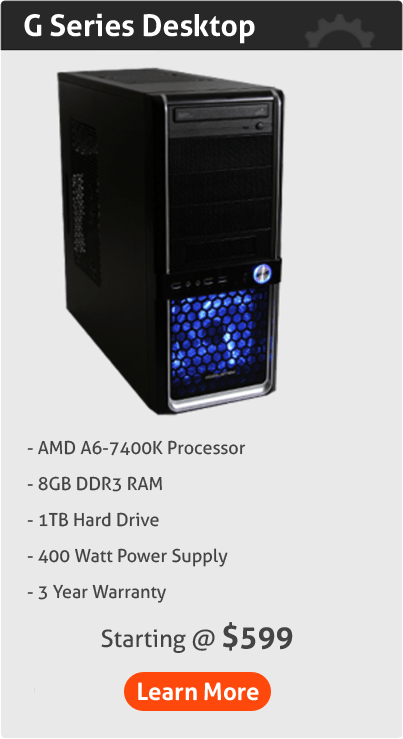This vintage magazine listing features a rectangular advert for the G-Series Desktop, presented vertically. At the top of the advertisement is a small section with a black background, showcasing the title "G-Series Desktop" in bold white letters. To the right of the title is the partial image of a gear in light gray, with its bottom portion cut off. 

Dominating the light gray background below is the image of a predominantly black computer tower. The bottom section of the tower features a square panel with a honeycomb pattern, illuminated by a bright blue light behind it. 

Beneath the tower image, a series of bullet points highlight the desktop's specifications: an AMD A6-7400K processor, 8GB DDR3 RAM, 1TB Hard Drive, 400W Power Supply, and a 3-Year Warranty. Centrally positioned on the page, it boldly states "Starting at $599."

At the very bottom of the advertisement, there's a horizontal, orange-colored bubble with the words "Learn More" inscribed in white, encouraging further engagement with the product.